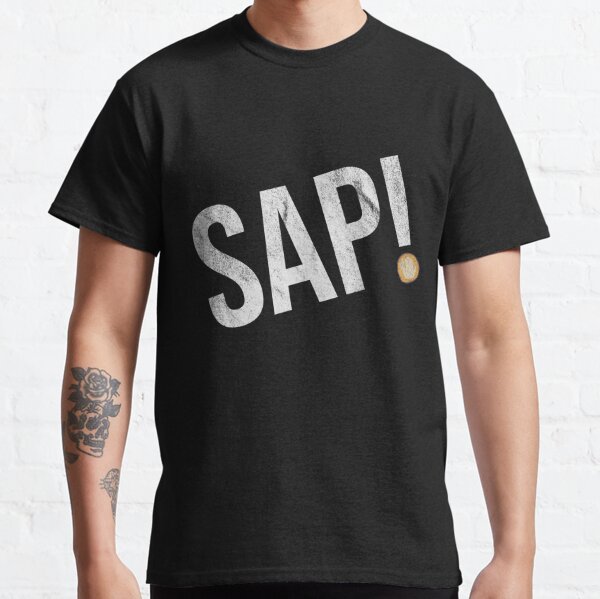In this close-up image, we see a male model from his neck down to just below his waist, showcasing a short-sleeved, black t-shirt. The shirt prominently features the word "SAP!" written in bold, all-caps, textured grey font with an exclamation mark. Notably, the dot of the exclamation mark is distinctly orange. The model's arms are positioned by his sides, revealing tattoos. On his right arm, towards the viewer's left, there is a detailed tattoo of roses with leaves, and another floral tattoo partially visible on his forearm. The background is completely white, accentuating the model's fair skin tone and the black t-shirt.